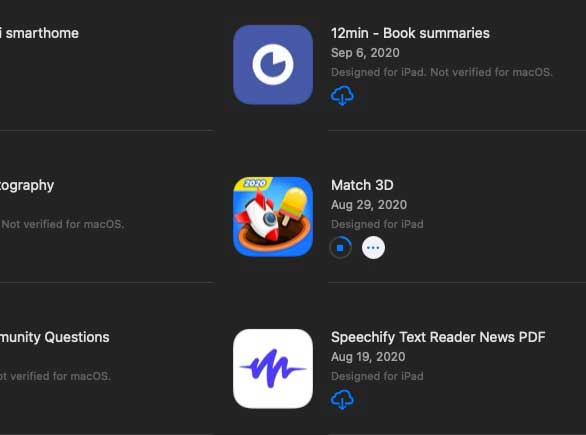On a solid black background, the left side of the image features white text somewhat obscured and incomplete. The decipherable portions of the text include phrases like "Smart Home," "O-G-R-A-P-H-Y," and "not verified for Mac OS." Additionally, there are mentions of "MUN," and what likely reads "Community Questions, verified for Mac OS." 

Centrally, the image showcases a column of app icons. The first icon has a blue background with a white circle, labeled "12-minute book summaries, September 6, 2020, designed for iPad, not verified for Mac OS," and noted as being stored in the cloud. 

Below it is the second icon, featuring an illustration of a spaceship and a popsicle, marked with "2020." This one reads, "Match 3D, August 29, 2020, designed for iPad," and is shown as currently downloading. 

At the bottom is a white square icon featuring a blue sound wave. It is identified as "Speechify Text Reader News PDF, August 19, 2020, designed for iPad," and indicated as being in the cloud.